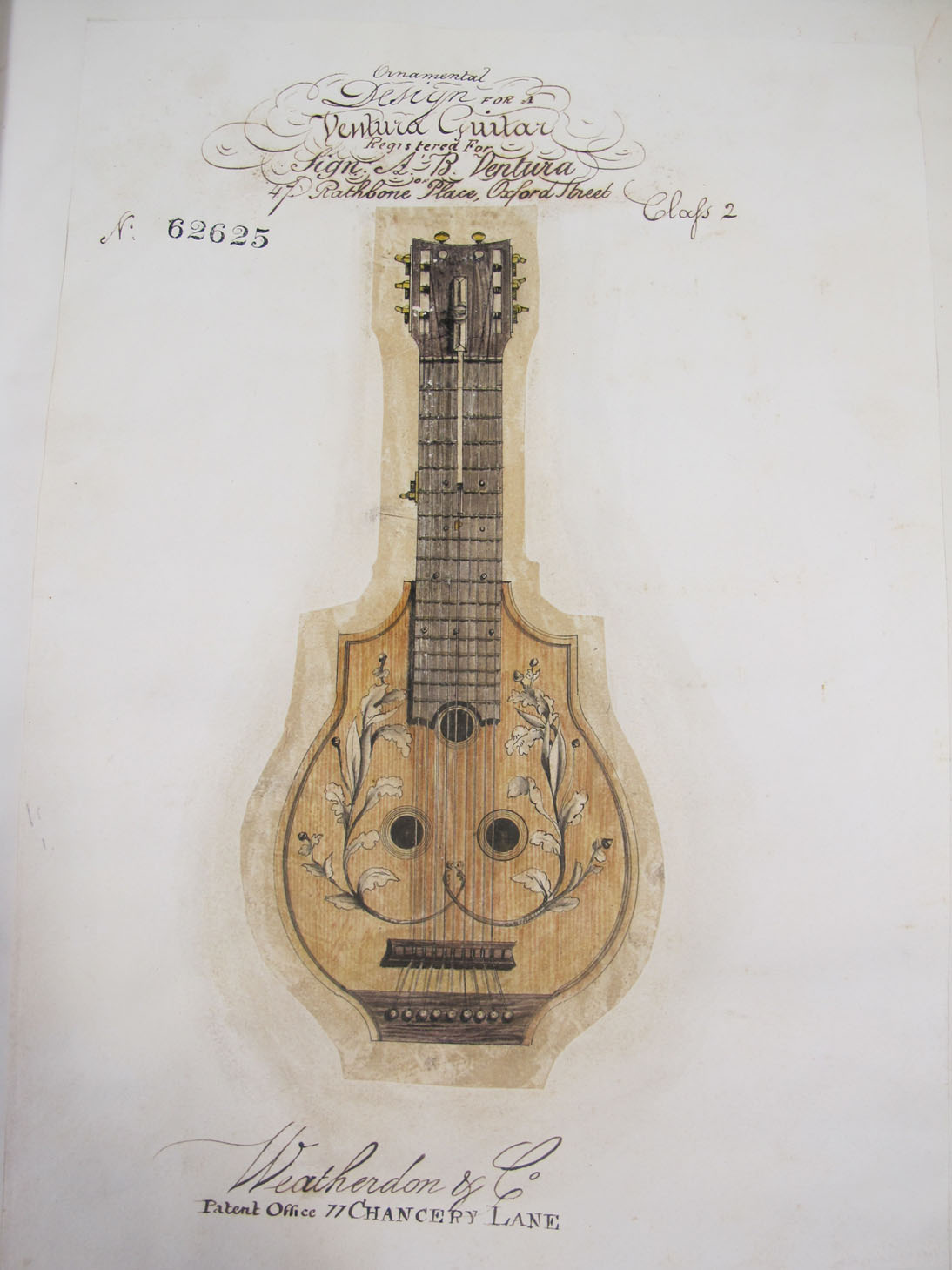This is a color photograph of an old illustration depicting a unique stringed instrument that closely resembles a hybrid between a guitar, a banjo, and possibly a lute or mandolin. The instrument, crafted from wood, features a distinctive design with three sound holes adorned with floral decorations, a short but thick double neck painted black, and a multitude of strings. The background of the illustration is an expansive white piece of paper, characterized by brown and pencil-colored sketches.

The top of the illustration displays stylized cursive text reading "Ventura Guitar," although parts of the script are difficult to decipher. Below this, there's a black ink stamp with the numbers "6-2-2-6-5." Additional text at the bottom reads "Weatherden and Company, Patent Office, 77 Chancery Lane," though there are variations in the readability of these elements across the captions.

Overall, the illustration combines artistic elegance with historical allure, capturing the intricate detailing and craftsmanship of the instrument and the accompanying ornate text.